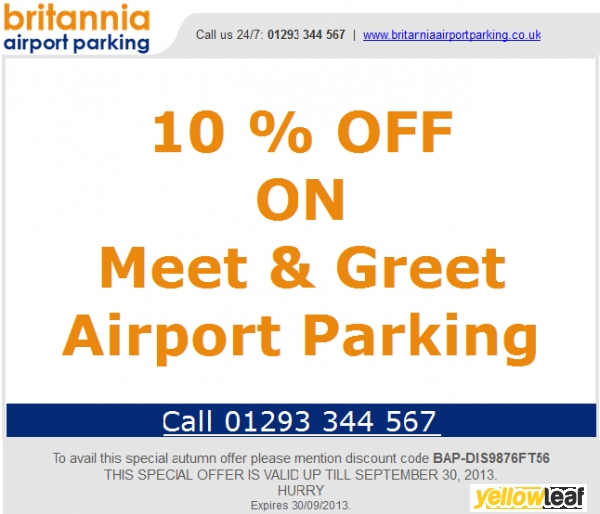This image appears to be a screen grab of an online advertisement for Britannia Airport Parking. The advertisement features a prominent offer displayed in the center. 

At the top left corner, there's the Britannia Airport Parking logo, featuring the words "Britannia" in orange and "Airport Parking" in blue. To the right, in a light gray box, there's a text instruction, "Call us at" followed by the phone number "01293 344567." A thin black line separates this from the next section.

Just below that, in blue text, the website address "www.britanniaairport.co.uk" is displayed. 

Dominating the middle of the screen, the main advertising message is shown in large, bold orange text: "10% off on Meet-and-Greet Airport Parking." 

Below this offer, inside a blue rectangular box, there's a call-to-action with the phone number "01293 344567" written in white text. 

At the bottom of the advertisement, in another light gray box, there's additional information: 

"To avail this special offer, please mention discount code BAP-DIS9876FT56. This special offer is valid up till September 30th, 2013. Hurry! Expires September 30th, 2013."

In the very bottom right-hand corner, there's a decorative yellow leaf with some text in yellow and black.

Overall, the advertisement is designed to grab attention with bold colors and clear, concise instructions on how to take advantage of the special offer.